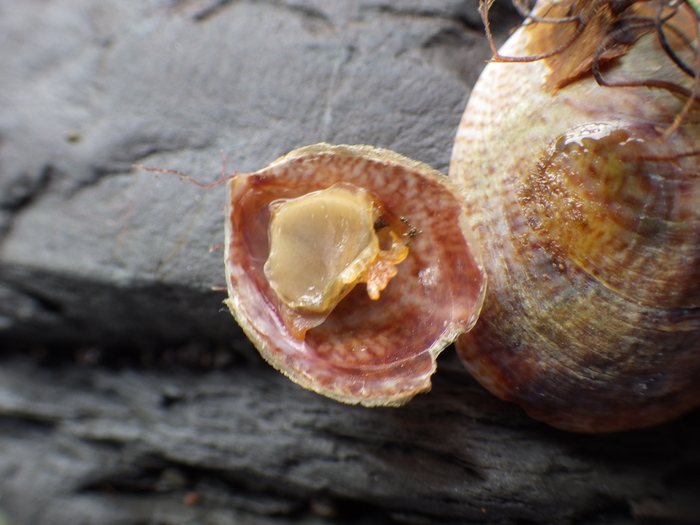This is a close-up color photograph of an open shellfish or mussel resting on a gray, rough stone surface. The stone appears slightly out of focus on the left side and looks like it could be petrified wood. The shellfish is opened wide, revealing its intricate details.

The base of the shell displays red and white bands with an amber hue, resembling veins spread across its surface. The inner part of the mollusk is visible; its oval-shaped, almost transparent, slimy body sits in the center, surrounded by a yellow rim. This body part has a hint of an amber tint underneath it. 

To the right, the photograph captures the top shell, characterized by a similar red and white banded pattern and featuring a large, slimy circle in the center. This part also has some orange specks on a white background. A few frail, amber-colored, hair-like structures extend from the top, adding to the delicate yet decayed appearance. 

Near the upper section of the image, you can spot some light brown, flat leaves, possibly seaweed, hanging down alongside the shell. The overall impression is that of a beautifully detailed, richly colored open shellfish perched on a naturally textured stone.